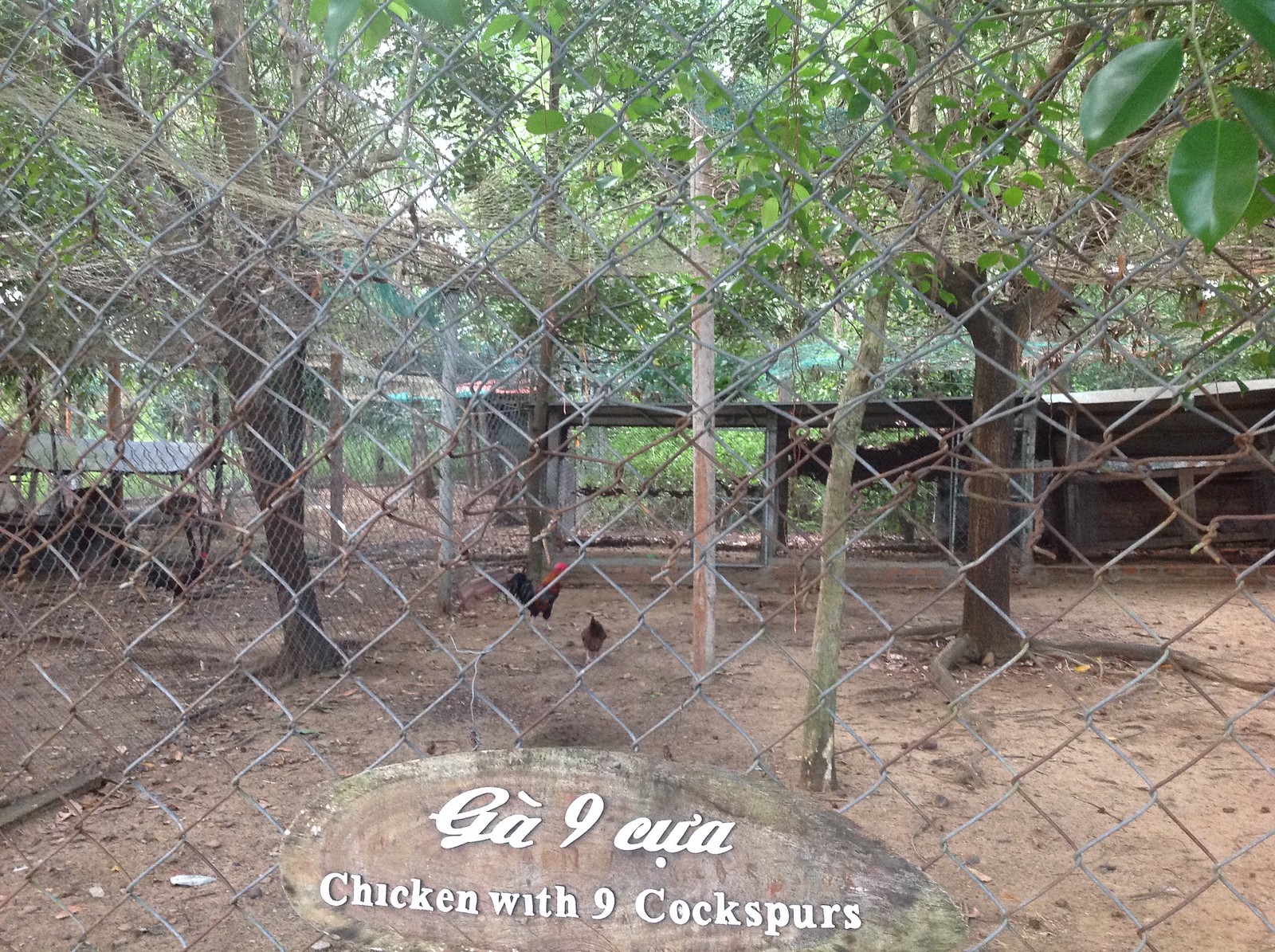This photograph captures a detailed and rustic view of a chicken enclosure situated outdoors, framed by a heavily rusted and distorted chain-link fence that twists in several places. The scene is abundant with lush greenery, featuring trees with verdant leaves both in the foreground and background. To the left side of the image, additional chain-link fences can be seen along with a large tree and several tree stumps scattered around. Inside the enclosure, there are visible chickens and roosters, with one prominent rooster and a smaller chicken closer to the fence. A weathered piece of wood, attached to the fence, displays text in white paint: "Gah 9 Kua" along with "Chicken with Nine Cock Spurs." In the background, man-made structures, possibly part of a chicken coop or additional roofing, are noticeable among the trees. Overall, this picture reveals a well-worn but lively habitat for the chickens, enclosed securely by extensive fencing.